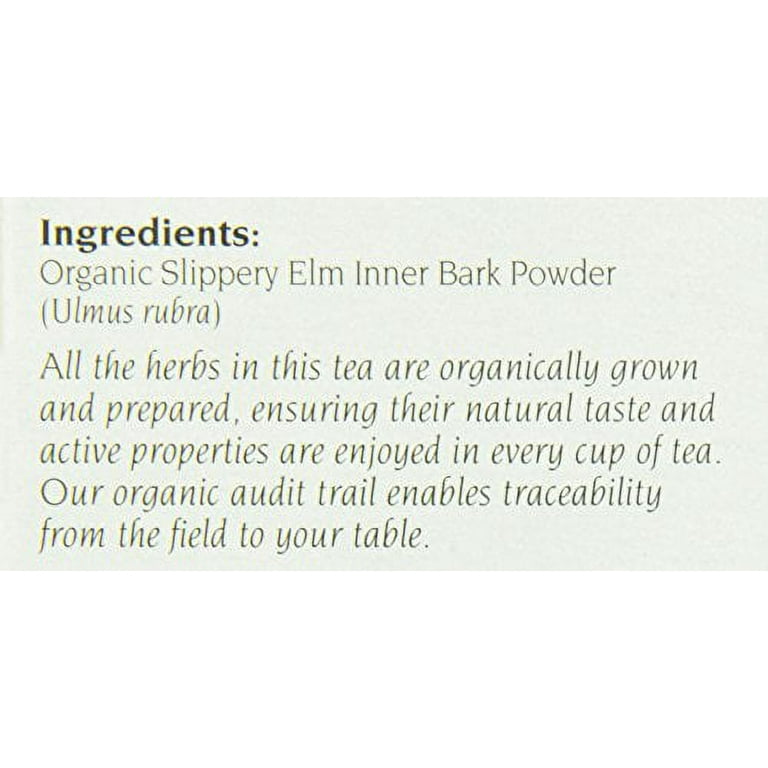The image features an ingredients label for a tea product printed on a pale sage green background. At the top left corner, the word "Ingredients:" is prominently displayed in bold, dark green font. Beneath this heading, it lists "Organic Slippery Elm Inner Bark Powder (Ulmus rubra)" in an easily readable, slightly fancy black text. The label further elaborates that "All the herbs in this tea are organically grown and prepared, ensuring their natural taste and active properties are enjoyed in every cup of tea." Additionally, the label highlights the brand's commitment to transparency with the statement, "Our organic audit trail enables traceability from the field to your table." This cohesive design employs a natural color palette and straightforward yet slightly elegant font, reinforcing the product's organic and healthful qualities.